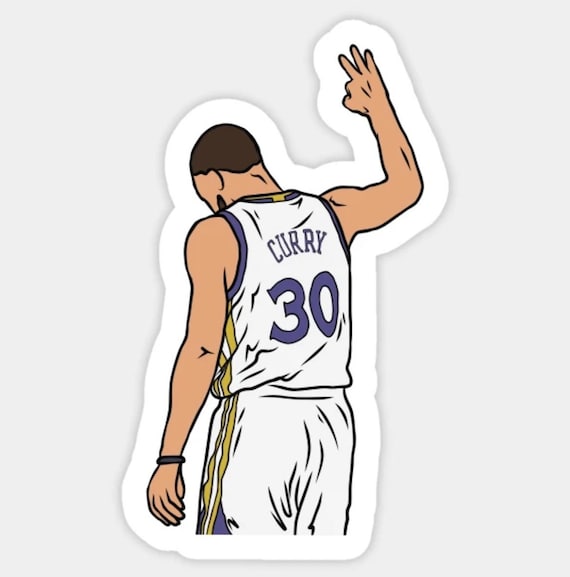The image depicts a detailed drawing of Steph Curry, the famous basketball player for the Golden State Warriors, rendered as a sticker or decal. The artwork is set against a layered background, with an outer light grey area and a white rectangle framing the drawing, which is predominantly blue. Curry is illustrated from the bottom of his shorts upwards, facing away from the viewer. He is wearing the Warriors' white jersey adorned with gold trimming along the sides, composed of two stripes, with additional blue and yellow elements. The name "Curry" is prominently displayed in blue block letters across his back, along with his iconic number "30." Curry's left arm hangs down by his side, equipped with a black wristband, while his right arm is raised to display three fingers, indicative of a successful three-pointer. His head is slightly bowed, adding a contemplative touch to the portrayal. The drawing captures the essence of Curry in his game-day attire, celebrating one of his many on-court achievements.